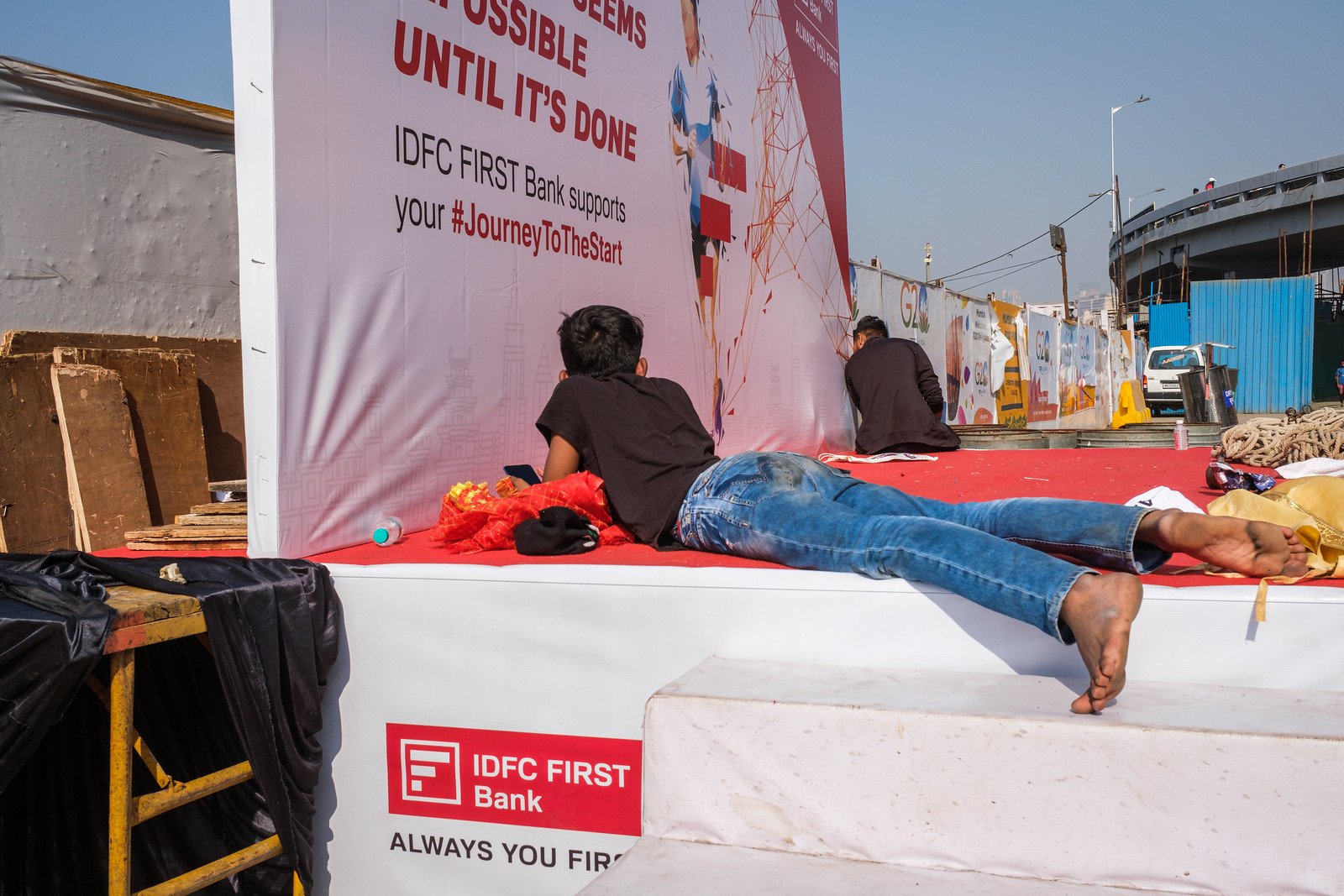In this detailed photograph, set in a bustling, urban environment that appears to be a modest part of town, two young men are positioned on a stage at an outdoor event. The stage, adorned with a red cloth and defined by white borders and stairs on the side, acts as a promotional platform for IDFC First Bank. The backdrop of the stage is a white banner with prominent red and black text that reads: "It seems possible until it's done. IDFC First Bank supports your journey to the start."

The foreground features a young man, approximately 10 to 18 years old, with light brown skin, dressed in blue jeans and a black short-sleeved shirt. He is lying on his stomach facing away from the camera, engrossed in his smartphone. Meanwhile, another man is seated on the opposite corner of the stage, also with his back turned towards us, appearing to focus on something in front of him, possibly painting or preparing the banner.

Beyond the stage, the city's structures, including a bridge, are faintly visible, enhancing the sense of a community-centered event set against a backdrop of daily life.